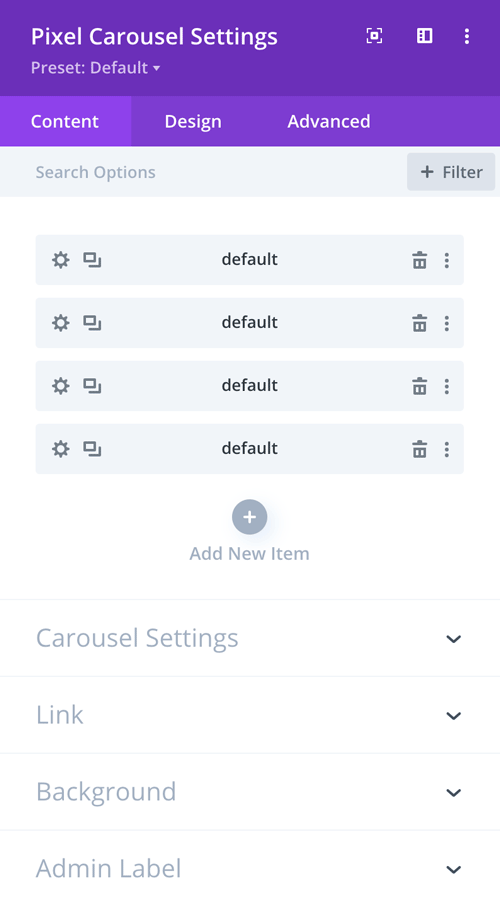The image depicts a screen capture of a mobile application interface. Dominating the top of the screen is a prominent blue banner displaying the title "Pixel Carousel Settings." Directly beneath this title, the text "Preset: Default" is visible, accompanied by a downward arrow indicating a dropdown menu.

In the upper right-hand corner of the blue banner, there are three vertical dots that reveal a secondary menu when tapped; adjacent to these dots is a notebook icon representing notes or documentation access.

Proceeding downward, the interface showcases a section with larger icons, including a picture icon, followed by three prominently labeled buttons against a lighter purple background: "Content," "Design," and "Advanced."

Below these buttons, a search bar labeled "Search Options" is presented, with a "Plus Filter" button situated to its right, presumably for adding search filters.

Further down, the screen is divided into four horizontal gray boxes, each containing a gear symbol (indicative of settings) and a rectangle symbol. Centrally within each box is the word "Default." To the right of these labels are a trash can icon, likely for deletion, and another set of three vertical dots for additional options.

Towards the bottom of the screen, a circular gray button with a plus sign inside invites users to "Add New Item."

Following this section, a series of expandable fields are shown, each with a downward arrow beside its label: "Carousel Settings," "Link," "Background," and "Admin Label," each designed to provide more options and configuration settings when tapped.

This detailed interface appears to offer extensive customization and settings options within the mobile application.